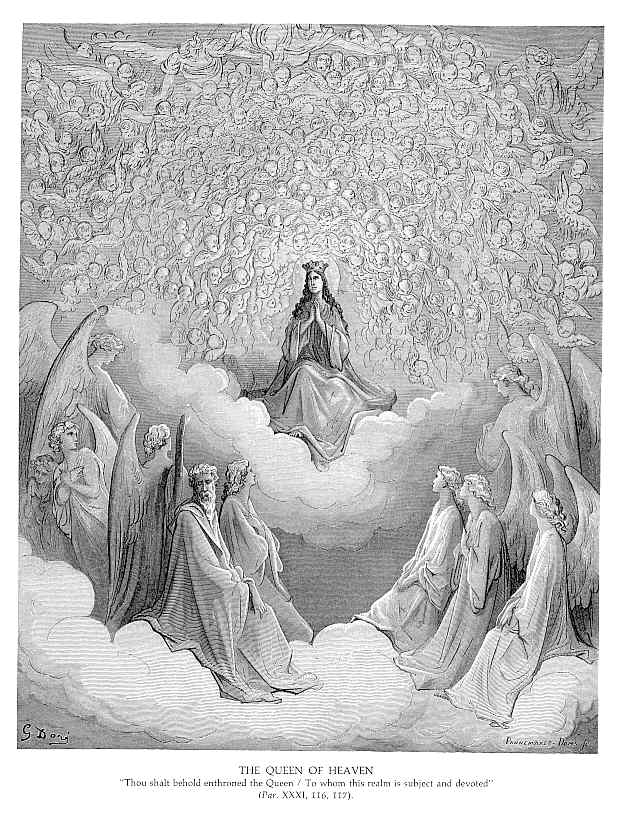The detailed black-and-white pen and ink drawing, attributed to Gustave Doré, depicts a figure identified as Mary, seated majestically on a cloud. Adorned with a crown and wearing a flowing robe, Mary is positioned centrally with her hands clasped in front of her. Surrounding her are numerous cherubic, Cupid-like angels behind her, while in the foreground, additional angels, some with wings, are kneeling and gazing reverently at her. These angels, along with a mix of possible gods and goddesses, are arranged on tiers of clouds, creating a divine and celestial atmosphere. Beneath this intricate scene, an inscription reads: "The Queen of Heaven, thou shalt behold and throne the Queen, to whom this realm is subject and devoted." The year is also indicated in Roman numerals, underscoring the engraving's historical and artistic significance.